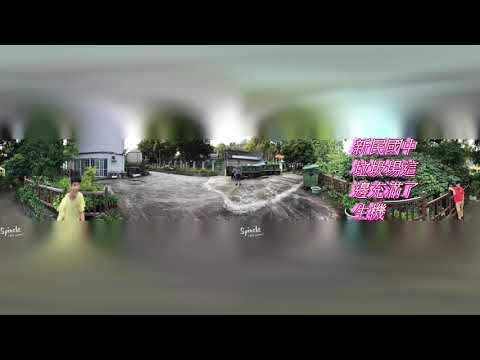This image depicts a somewhat blurred outdoor street scene, possibly a photograph or digitally generated image with a fisheye effect. The central horizontal band of the image is the clearest, flanked above and below by glassy, blurred sections, with horizontal black bars further accentuating the top and bottom. 

In the scene, a white house with sliding doors and grid-style windows can be seen in the background on the left. The ground of the walking path is characterized by a dark color interspersed with white spots, bordered by a wooden, brown fence entwined with vines. Trees and green plants adorn the side of this path.

Towards the right side, pink Asian characters, possibly Chinese or Japanese, are visible. Two figures are present: one person in a light green or yellow shirt with short black hair stands near the center, while another, wearing a red shirt and khaki pants, is leaning against a fence or walking or riding a bicycle. Additional elements in the scene include a green dumpster and what appears to be a dirt path leading up to the house.